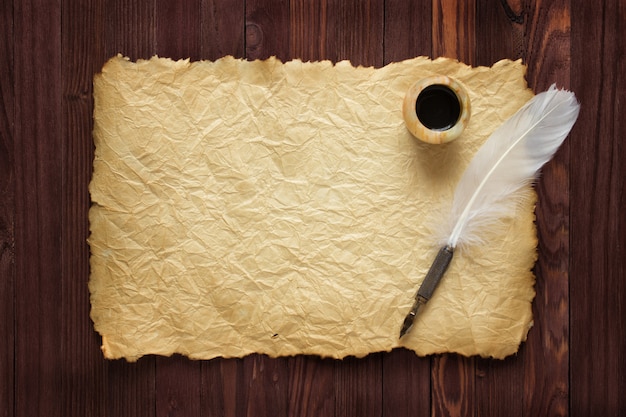The image showcases an overhead view of a dark mahogany wooden table with rich, honey-hued grain and knots. Resting on the table is a weathered piece of parchment paper, characterized by its crinkled, yellowish surface and frayed, uneven edges suggesting an antiquated or historic appearance. On this parchment lies a white feather pen with a metal handle and nib, poised towards the lower left of the image. The pen, featuring some form of leather binding, remains untouched and ready for use. Beside it, partly weighing down the parchment, is a round, marble-finished ink bottle containing black ink, its beige and darker beige splotched surface almost blending with the parchment itself. The composition evokes an old-school script setup, meticulously posed to highlight the anachronistic charm of traditional writing instruments.